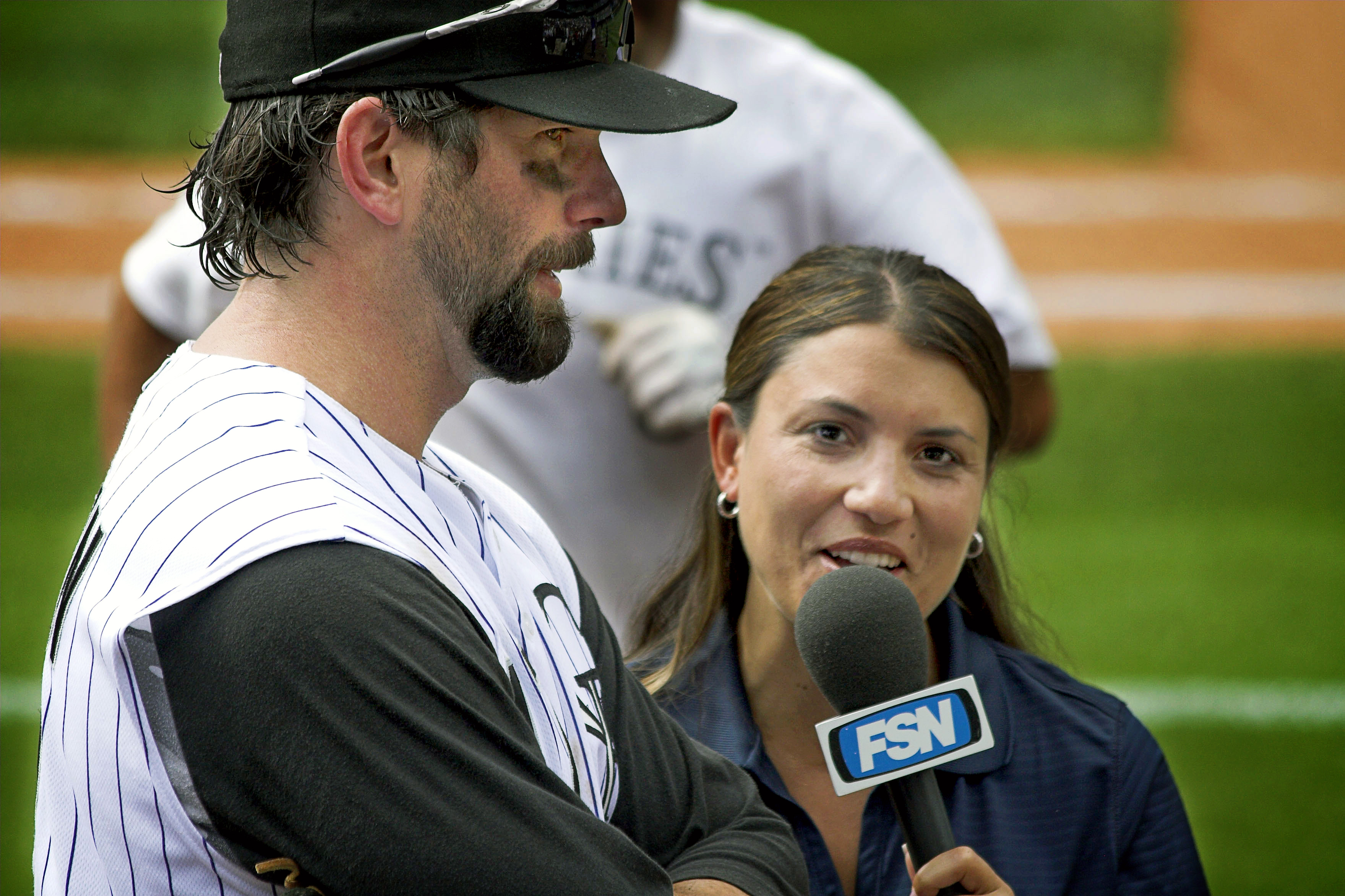In the image, a bearded baseball player with long black hair, wearing a white jersey with black pinstripes over a black long-sleeved shirt, stands with his arms folded. He sports black eye smudges, a black hat with silver sunglasses perched on top, and a sweaty appearance. He's being interviewed on the field by a Latina woman in her 40s, who has long brown hair and is dressed in a blue outfit with silver hoop earrings. She holds a microphone labeled FSN and smiles at the camera. In the background, you can see the green grass, the baseball diamond with brown dirt and white lines, and another player in a white t-shirt and white gloves running towards them.